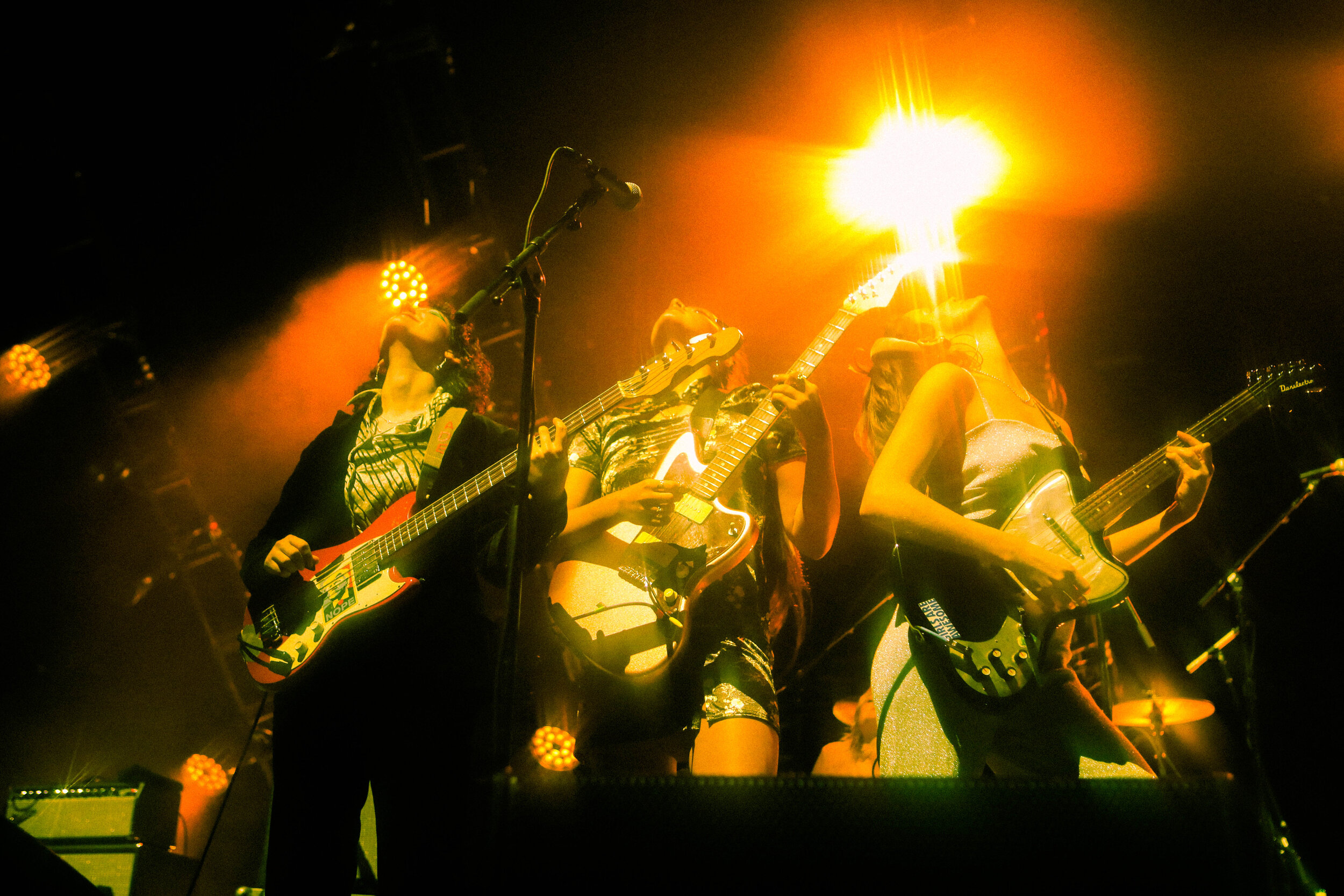This photograph captures an all-girl band performing live on stage from an audience perspective. The image is taken from right in front of the stage, looking up at the three women, each playing an electric guitar. Notably, all three musicians are gazing upward, though it's unclear what they are looking at. The background is enveloped in darkness, accentuated by a bright stage light that creates a smoky ambiance, highlighting the outlines of the smoke around the light. Each band member is distinctly dressed: the woman on the far left is in black, the middle musician sports a striped t-shirt, and the woman on the right wears a halter top. Additional stage elements include a microphone stand aimed at the middle musician and various equipment like an amp and more lights, including one with dotted edges above the middle guitarist. The image effectively conveys the intensity of a live performance, with the stage and its details vividly captured.